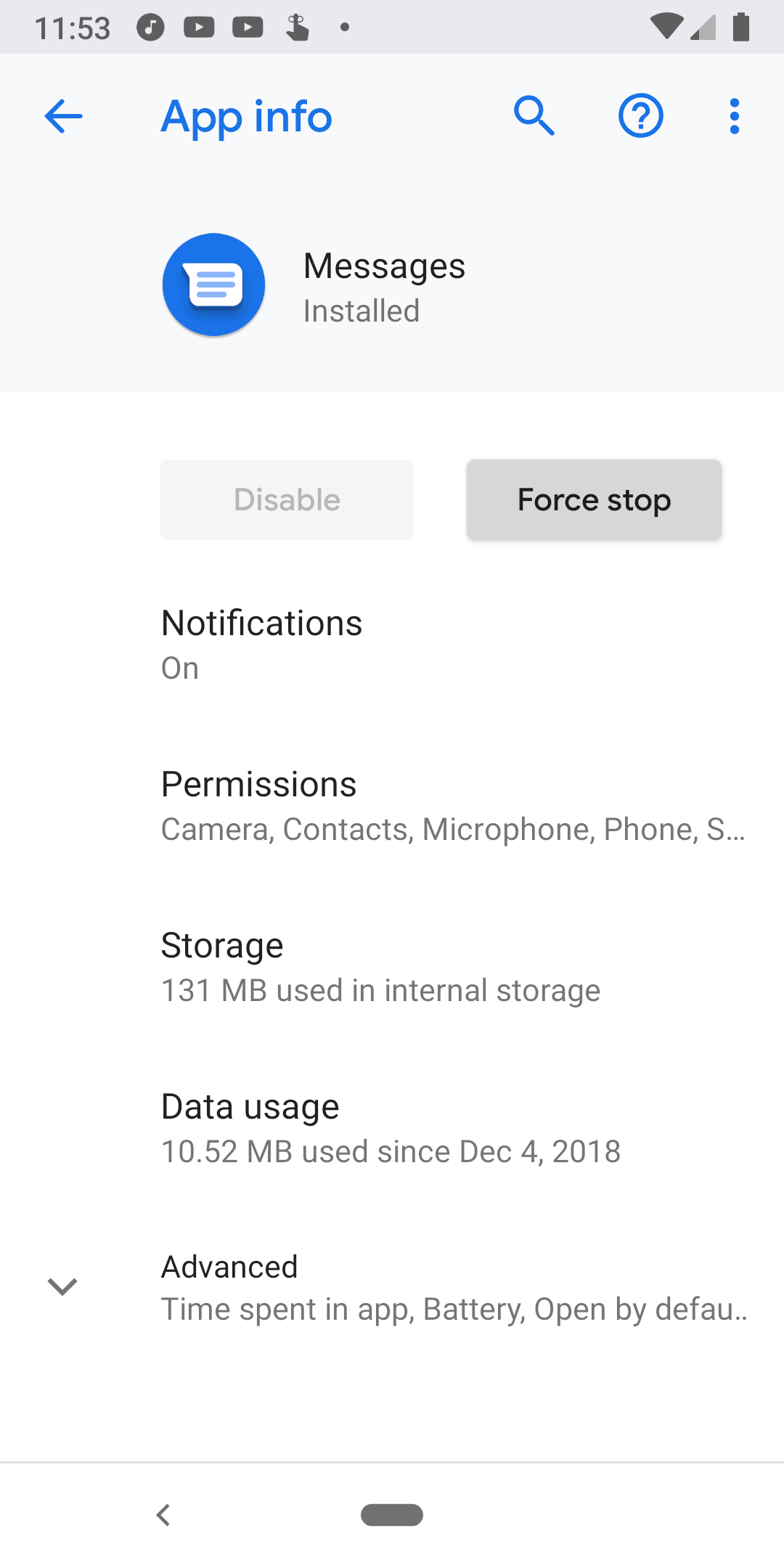The image appears to be a screenshot of someone's smartphone displaying the "App Info" page for the Messages application. The screenshot is identifiable by its rectangular shape with a predominantly white background. 

In the top right corner, typical phone status indicators are visible, including icons for Wi-Fi, cellular signal strength, and battery level. The time is displayed in the upper left corner, showing "11:53," alongside other common smartphone symbols.

Beneath a light blue header labeled "App Info," the Messages app icon is displayed within a blue circle, accompanied by the text "Messages" and the note "Installed."

Below this, there are two options: "Disable" and "Force Stop." The "Disable" button is rendered in a very light gray color, suggesting it is not selectable, while "Force Stop" is displayed in dark gray with black text, indicating it is available for selection. 

Further details listed include:
- "Notifications: On"
- "Permissions: Camera, Contacts, Microphone, Phone, ...," with the list truncated, indicated by an ellipsis.

Following permissions, the storage information reads "131 MB used in internal storage." Data usage since December 4, 2018, is noted as "10.52 MB."

Next, under "Advanced," it mentions "Time spent in app," "Battery," and "Open by default." 

The screenshot ends here with no additional information visible about the app, which is identified as the standard Messages app used for texting and communication on the device.